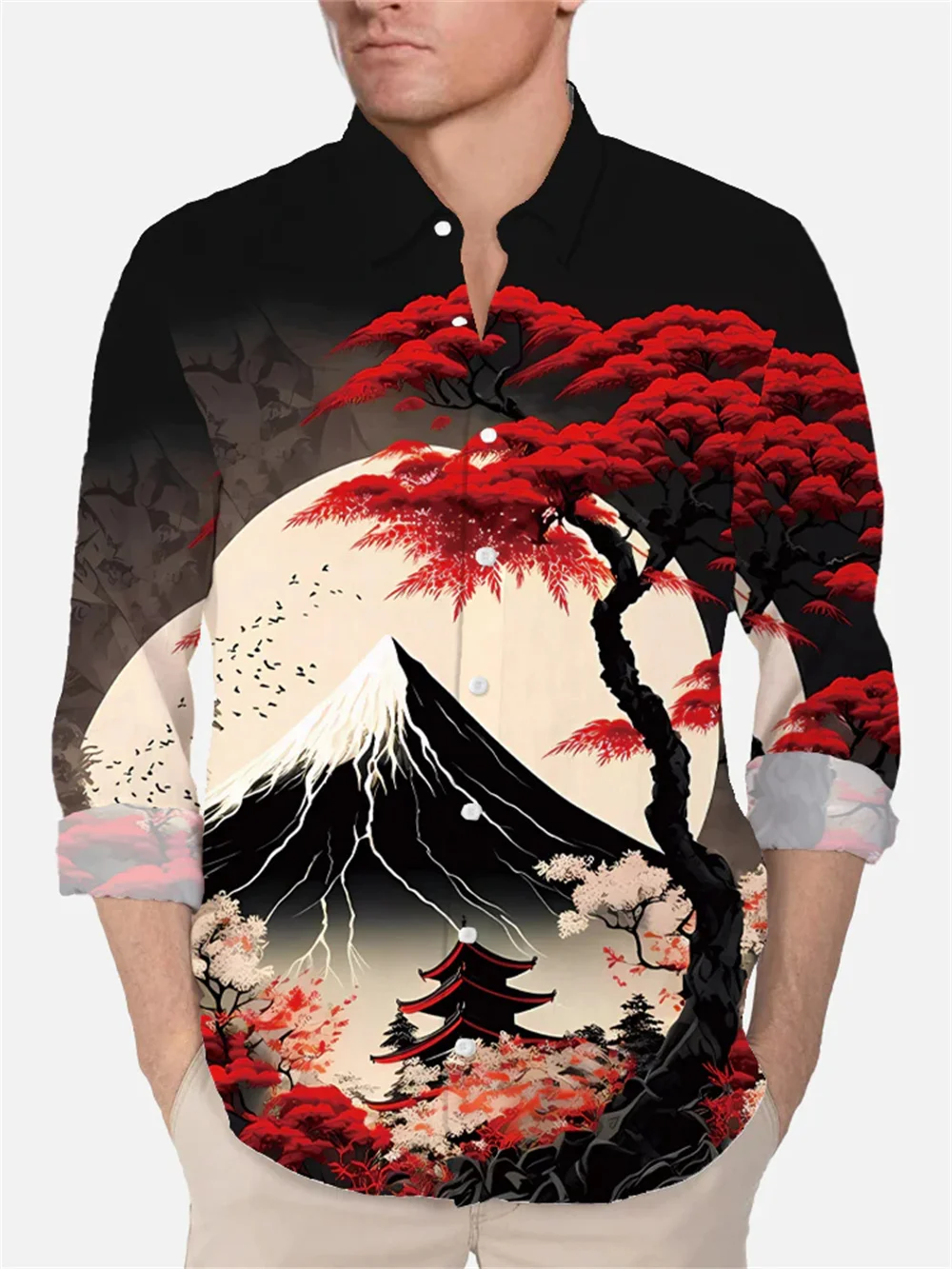The photograph captures a man from the nose down to just above the thighs, set against a white background, suggesting it might be an advertisement for the shirt he’s wearing. The man sports a slightly unhappy, neutral expression. The shirt is a long-sleeved, cotton button-down with the sleeves folded up below the elbow, featuring a detailed, Asian-inspired design. The upper part of the shirt, including the collar, is black with white buttons. The bottom showcases a striking scene on a black background, dominated by a massive white moon spanning the shirt's width. 

In the foreground, a large, black-silhouetted tree with vibrant red leaves extends upwards, with the branches nearly reaching the man's throat and spreading down one sleeve. The scene includes a towering, black silhouetted mountain with distinctive white details and a cracked texture, suggesting ice, snow, and rivulets of water. Below the mountain sits a Japanese-style temple or pagoda with a spire and red lining on the roof, flanked by red and white cherry blossom trees. Additionally, a flock of birds is flying to the left of the mountain. The man's lower half is adorned with plain khaki pants, effectively allowing the intricate artwork of the shirt to be the focal point.